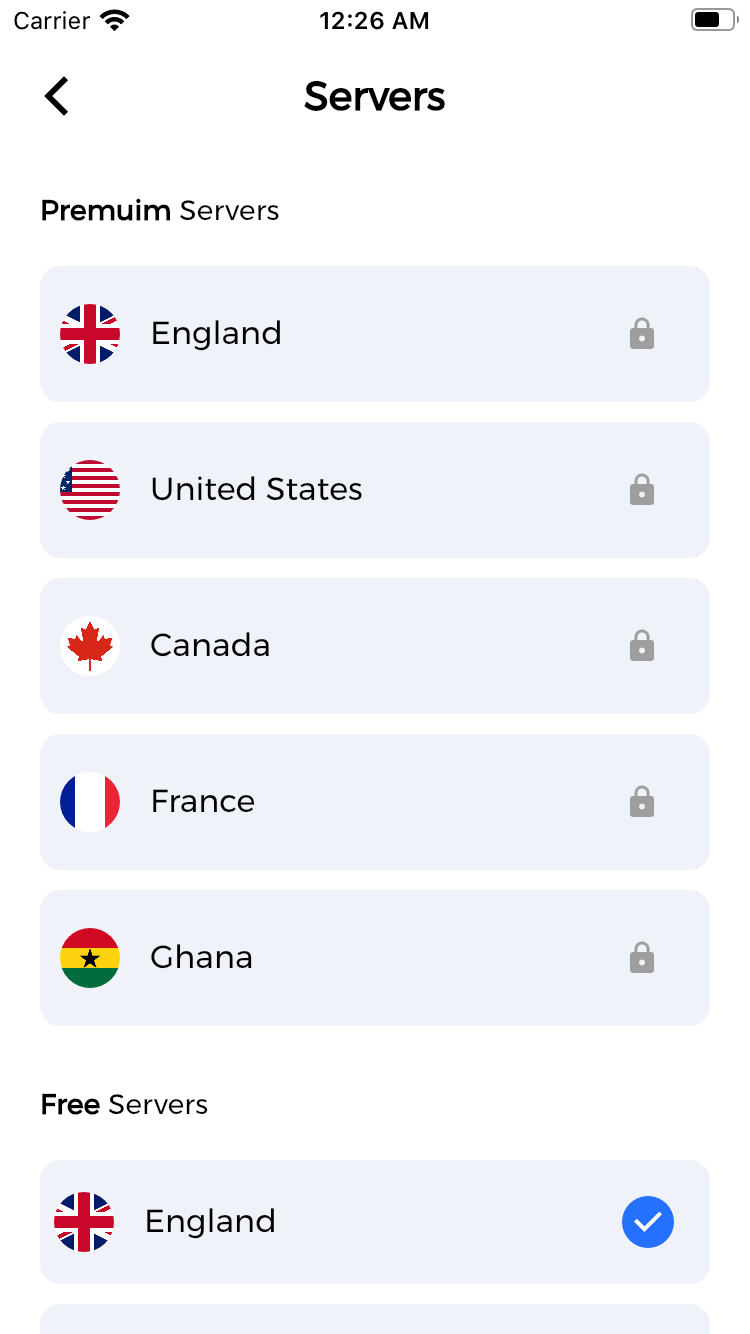This mobile screenshot, oriented vertically, displays the interface of an app. The top left corner shows the "Carrier" label alongside the black Wi-Fi icon, and the time reads 12:26 AM. In the top right corner, the battery icon is approximately 70% full. Below the time, the word "Servers" is displayed with a left-pointing arrow indicating navigation options.

Underneath "Servers," the title "PREMUIUM SERVERS" is prominently featured, albeit with a typographical error ("premium" is misspelled as "premuim"). The section contains five light blue horizontal bars, each listing a different country with corresponding elements. On the left of each bar is a circle displaying part of the country’s flag; on the right is a gray lock icon.

- The first bar is labeled "England," showcasing the English flag with its iconic red cross on a white background, and a blue background with white and red elements.
- The second bar represents the "United States," featuring alternating red and white stripes with a fragment of the blue field containing white stars.
- The third bar is labeled "Canada," depicted by the white background and red maple leaf of the Canadian flag.
- The fourth bar is "France," represented by vertical stripes of blue, white, and red.
- The fifth bar is "Ghana," showing horizontal stripes of red, yellow, and green with a black star in the center.

Below these "PREMUIUM SERVERS," the section titled "Free Service" features "England" again, displaying the UK flag with an additional blue check mark on the right, indicating selection or active status.